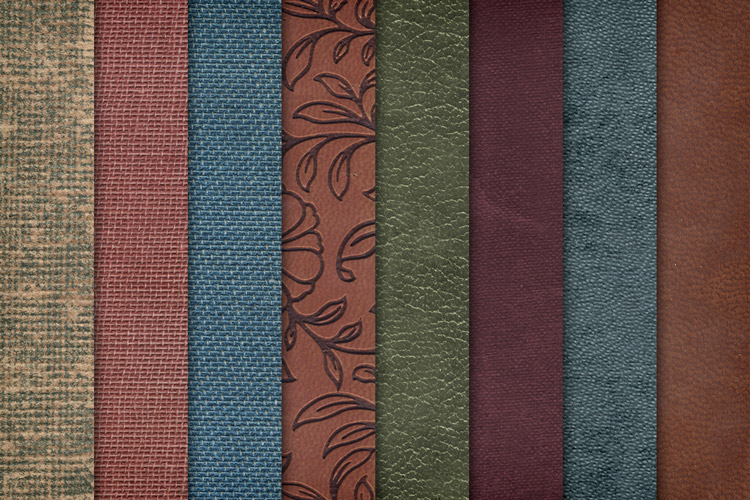The image shows eight vertically aligned, narrow rectangular strips of fabric laid out evenly from left to right. Each strip features a different color and texture, ranging from green, tan, light red, light blue, brown with floral patterns, dark green, magenta, bluish-green, to brown suede. The arrangement includes overlapping sections, adding visual depth and texture contrast. The brown strip in the center is especially notable for its decorated leaves and floral patterns, possibly indicating a leather material. This detailed fabric assortment showcases unique styles and colors, such as a green leather-textured strip, a burgundy one, and another brown strip resembling suede, effectively demonstrating the variety of fabrics available.